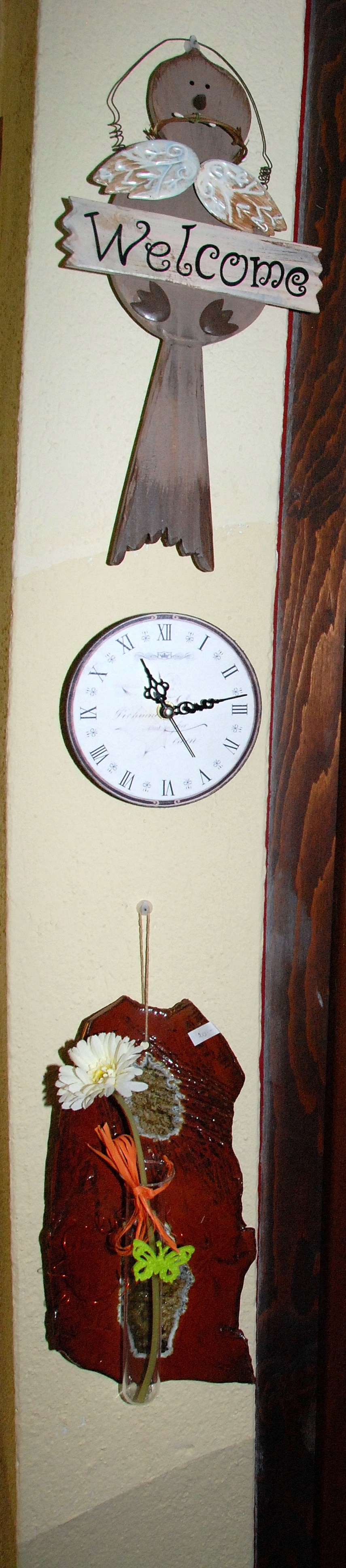The image depicts a section of an interior wall, possibly a soffit, painted in a soft tan color. Adorning this wall are three distinct decorations. 

At the top hangs a charming wooden sign taking the shape of a whimsical bird. The bird is predominantly brown with white wings, a long tail, and cute webbed feet, all lending it a playful appearance. The bird's face and feet are black, and it holds a small wire for hanging. Across its midsection, a black "Welcome" message is printed on a plaque running horizontally across the bird's body.

Positioned below the bird is an elegant round clock with a classic white face and black Roman numerals. The clock shows the time as 11:13, and its hands are designed to resemble gear keys, with a second hand completing its functionality. Notably, the Roman numerals for four through eight are positioned upside down, adding a unique touch to its design.

At the bottom of the arrangement, a wooden plaque decorated with motifs of nature adds a touch of rustic charm. The plaque features a white daisy, strands of orange yarn, and a green butterfly, creating a simple yet pleasing floral scene.

This trio of decorative elements brings a homely and welcoming feel to the wall, combining functionality with aesthetic appeal.